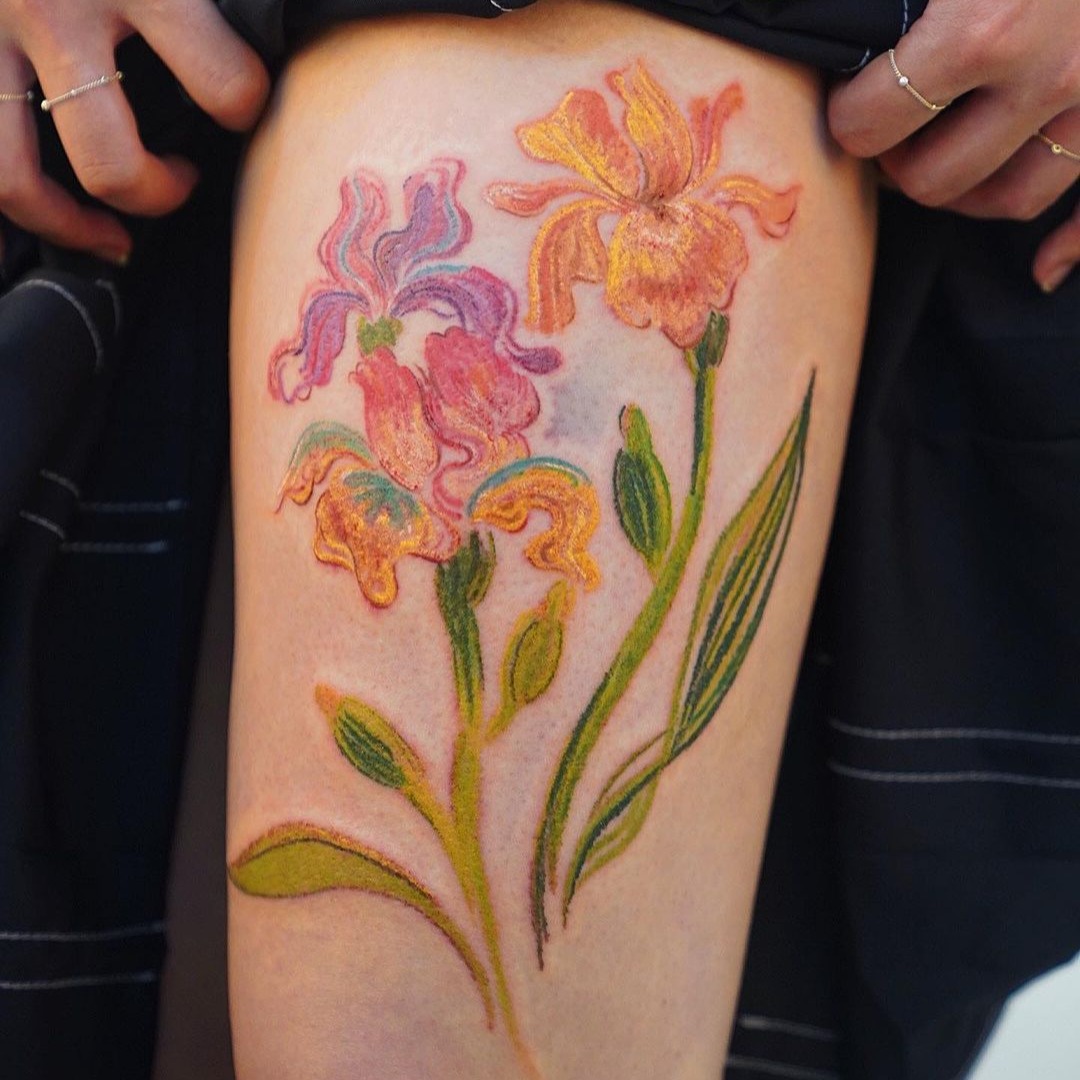This detailed, square photograph, approximately 6 inches by 6 inches, captures the front thigh of a Caucasian woman's leg, adorned with vibrant tattoos. The woman, seen from the waist down, is using her left and right hands – emerging from the upper left and right corners of the image – to pull up the dark blue hem of her skirt, revealing intricate floral body art. Her slender fingers are decorated with thin silver rings on her forefinger, ring finger, and middle finger.

The tattoos depict two vividly colored iris flowers with long green stems, each with distinctive hues and detailed design. The stem on the left starts with a lighter green at the base and transitions into a darker green, leading up to an iris with pink petals accented by blue and yellow highlights. Behind it, there is a secondary bloom in shades of blue and purple, without a visible stem. Meanwhile, the stem on the right is a darker shade of green from the start and supports a flower with petals that blend yellow, pink, and touches of green, giving an impression of a hand-colored sketch. This rich, dynamic artwork vividly showcases the woman’s unique and colorful tattoos.